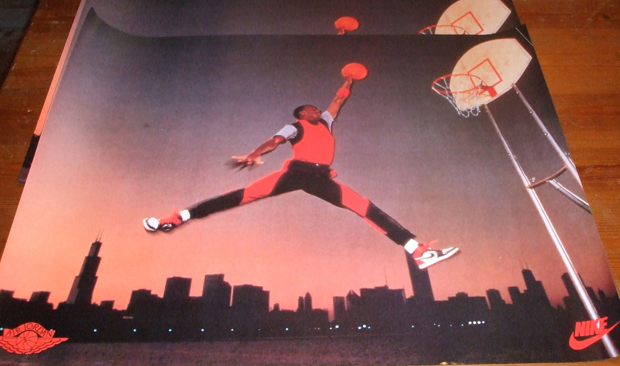The image is a color photograph of a retro Nike advertisement poster featuring Michael Jordan performing his iconic dunk. Centered in the frame, Jordan soars mid-air, legs spread wide, about to slam a red basketball into a white hoop with a visible square backboard and nylon net. He wears a distinctive red and black uniform with a black and red tank top, gray sleeves, and matching pants, accented by his famous Air Jordan sneakers in red, black, and white. The backdrop of the poster showcases the silhouette of the New York City skyline, suggesting an outdoor nighttime setting. The print, resting on a wooden table, also includes the Nike logo prominently in the lower right corner, adding a classic touch to the vintage athletic advertisement.